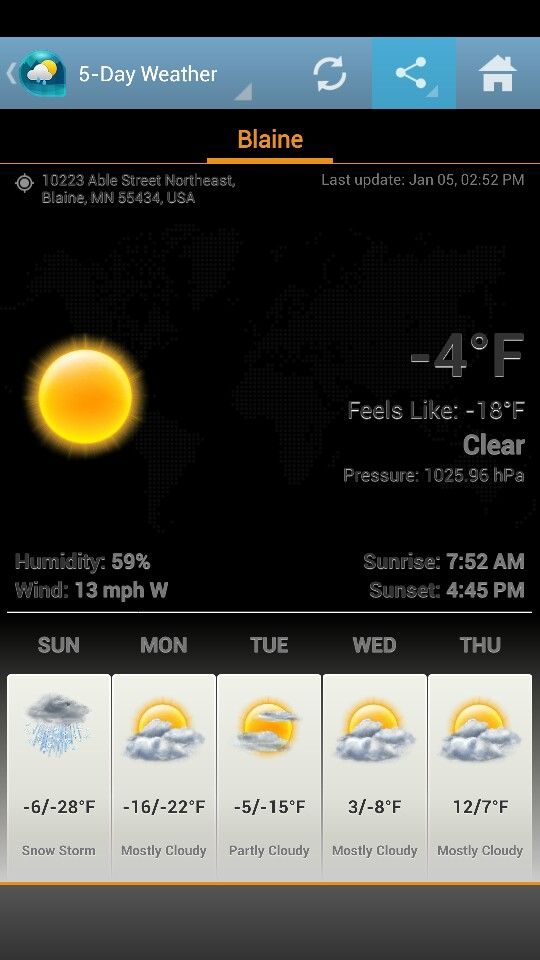This is a detailed screenshot from a mobile weather app, capturing the weather report for Blaine, Minnesota. The app's interface features a black banner at the top, followed by a blue banner that displays the app's logo and the text "5 Day Weather." Alongside this, there are three utility icons: a refresh icon, a share icon, and a home icon.

The location, "Blaine," is prominently displayed in orange lettering, indicating the city for the weather report. Beneath this, the exact location is specified as 10223 Abel Street, North East Blaine, MN 55434, USA. The report provides the latest update timestamped at January 5th, 2:52 PM.

The background is black, and on the left side, a blazing sun icon indicates clear conditions. The detailed weather data includes 59% humidity and a wind speed of 13 miles per hour from the west. On the right side, in large font, the temperature is shown as -4°F, with a "feels like" temperature of -18°F. The pressure is recorded at 1025.95 HPA. The sunrise is at 7:52 AM, and the sunset is at 4:45 PM.

Below this, five tiles represent the upcoming days, each labeled with the day of the week—Sunday, Monday, Tuesday, Wednesday, and Thursday. Weather icons illustrate the forecast for each day: Sunday is stormy, Monday is partly sunny and cloudy, Tuesday is mostly sunny with slight clouds, and both Wednesday and Thursday are partly sunny and cloudy.